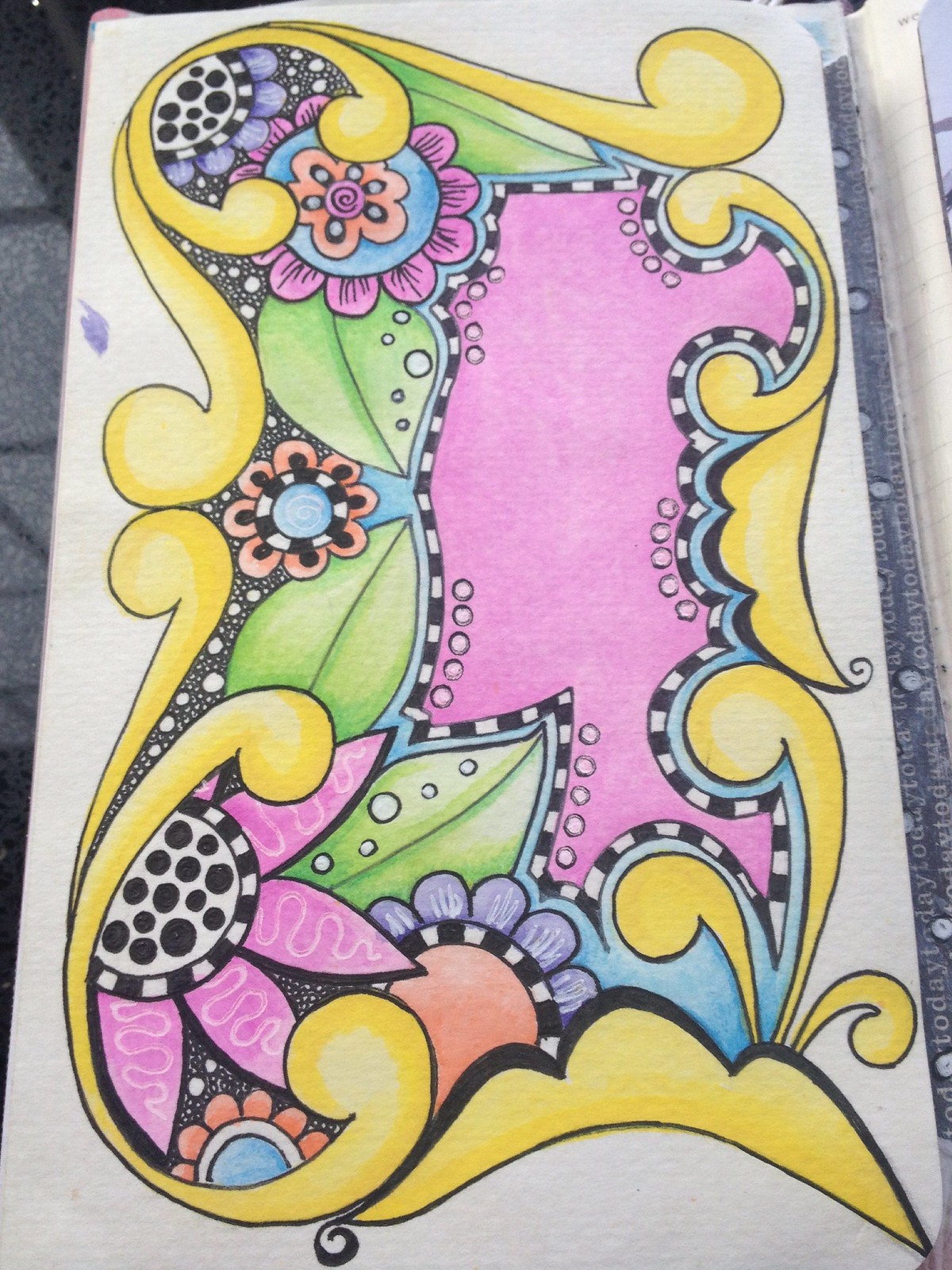The image features a vibrant, abstract artwork on a large, rectangular white canvas, likely created with crayon or colored pencils. The composition is adorned with looping, yellow apostrophe-like scrolls that form a border. Within this border, a series of flowers and leaves are intricately illustrated. The flowers showcase a variety of colors including pink, purple, orange, blue, green, black, and white. Specifically, some flowers have blue centers paired with pink petals, others feature alternating black and white rings around blue centers with different combinations of orange, pink, and purple petals. There is also a standout flower with a white background, black dots, and pink petals. The artwork includes four distinct green leaves and some pieces resembling puzzle shapes highlighted in pink. Additionally, a large central purple area occupies the middle of the canvas. The background behind the artwork is dark and indeterminate, possibly dark blue, leaving the setting ambiguous.